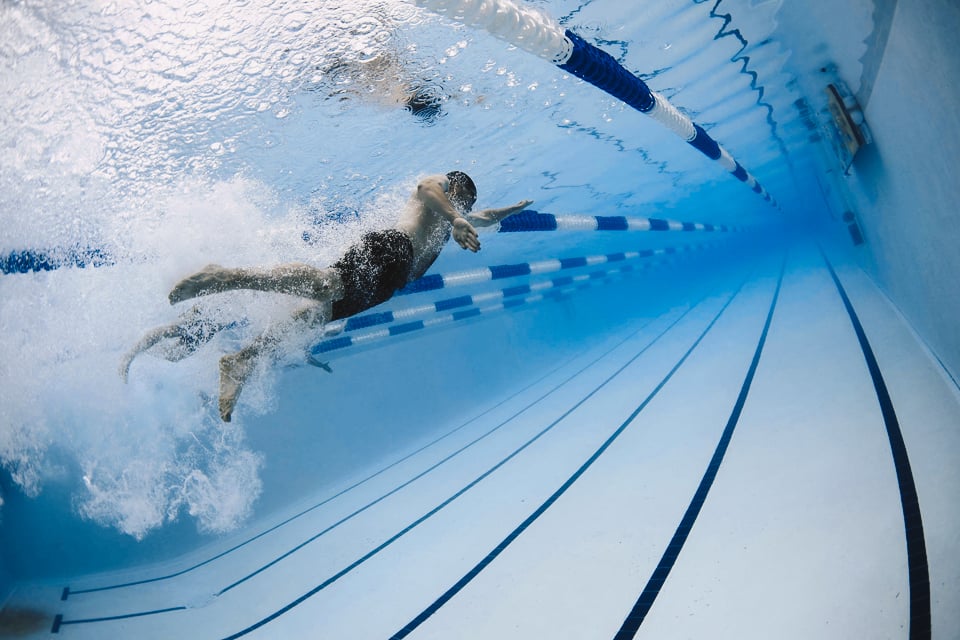This underwater photograph captures the interior of a long, lap-style swimming pool. As we view the scene from the back corner, the white pool floor is clearly marked by long black lines that run its length, ensuring swimmers stay within their lanes. Above, white and blue buoy-style ropes stretch across the surface, effectively separating the lanes. The water’s color transitions from a clear, lighter blue near the foreground to a darker blue as it moves towards the far end. Along the left side of the image, two swimmers clad in black trunks are in motion, creating a flurry of white bubbles and ripples with their kicks. The photograph suggests the swimmers might be practicing for a competition, given their focused movements and the structured layout of the pool.